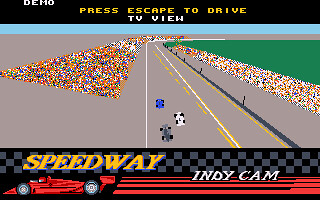The image depicts a retro-style video game interface featuring a high-speed racing scene. At the top, a blue stripe displays the words "Demo" in white, "Press Esc to Drive" in yellow, and "TV View" in white. At the bottom, another stripe reads "Speedway Indy Cam" in white text. The focal point is a red Indy race car, positioned on the left side of the image, with dynamic motion trails suggesting it's speeding across the screen.

The race track takes up the central part of the screen, bordered by what appears to be a colorful, pixelated crowd on both the left and right sides. A green triangular section on the right simulates grass, while two gray stripes represent different parts of the race track. A lane featuring a dotted yellow line and a solid yellow line runs through the scene. Three additional race cars—a blue one, a white one slightly to the right, and a gray one nearly parallel to the blue car—are also visible. Black wheels are noticeable on all cars. Above the cars is a checkerboard pattern beneath the word "Speedway," which is written in yellow. The section labeled "Indy Cam" in white is displayed against the blue background. The entire scene conveys the excitement of an intense race in progress.